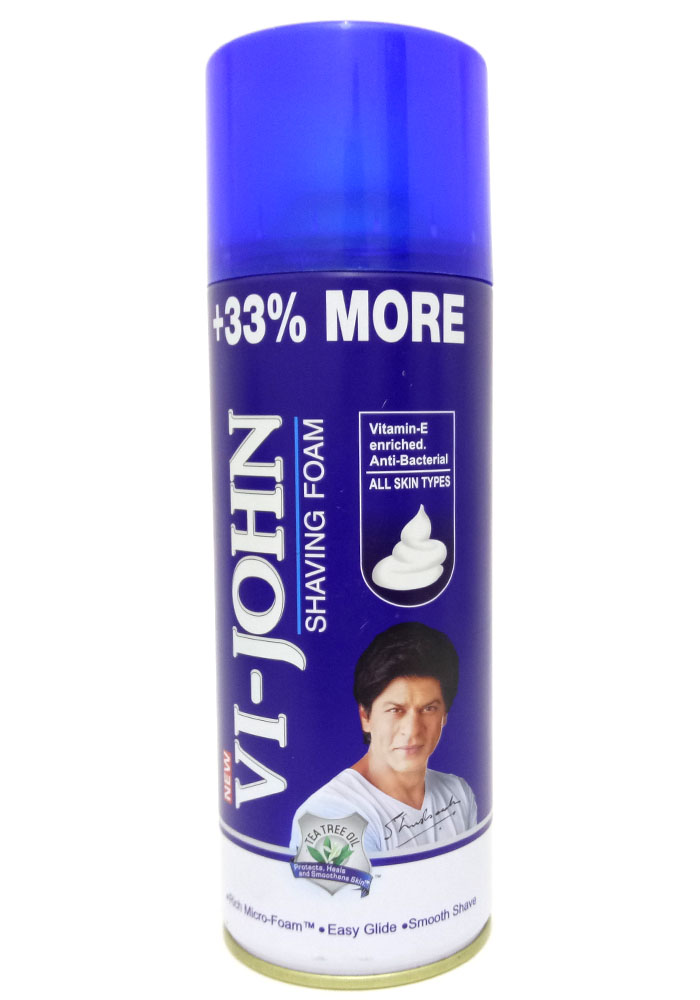This image showcases a tall, cylindrical can of shaving foam with a blue metal body and a matching blue plastic lid. Directly beneath the lid, the can prominently displays the text "Plus 33% More," indicating a larger-than-standard size. Vertically aligned along the can's body is the brand name "VI-John" in large, 3D-effect white letters. Below this, another vertical line of text reads "Shaving Foam," separated by a light blue line. Adjacent to this sequence, various product features are highlighted, including "Vitamin E Enriched," "Antibacterial," and "For All Skin Types." There is also an image illustrating the foam texture. Toward the bottom of the can, there is a photograph of a man with thick black hair, olive skin, and wearing a white t-shirt, accompanied by his signature. Around his portrait, a silver sheriff's badge symbol contains the text "Tea Tree Oil." At the base of the can, a series of product benefits are listed in blue text, separated by small dots: "Rich Microfoam™," "Easy Glide," and "Smooth Shave." The can rests on a gold-colored base, adding a touch of elegance to its design.